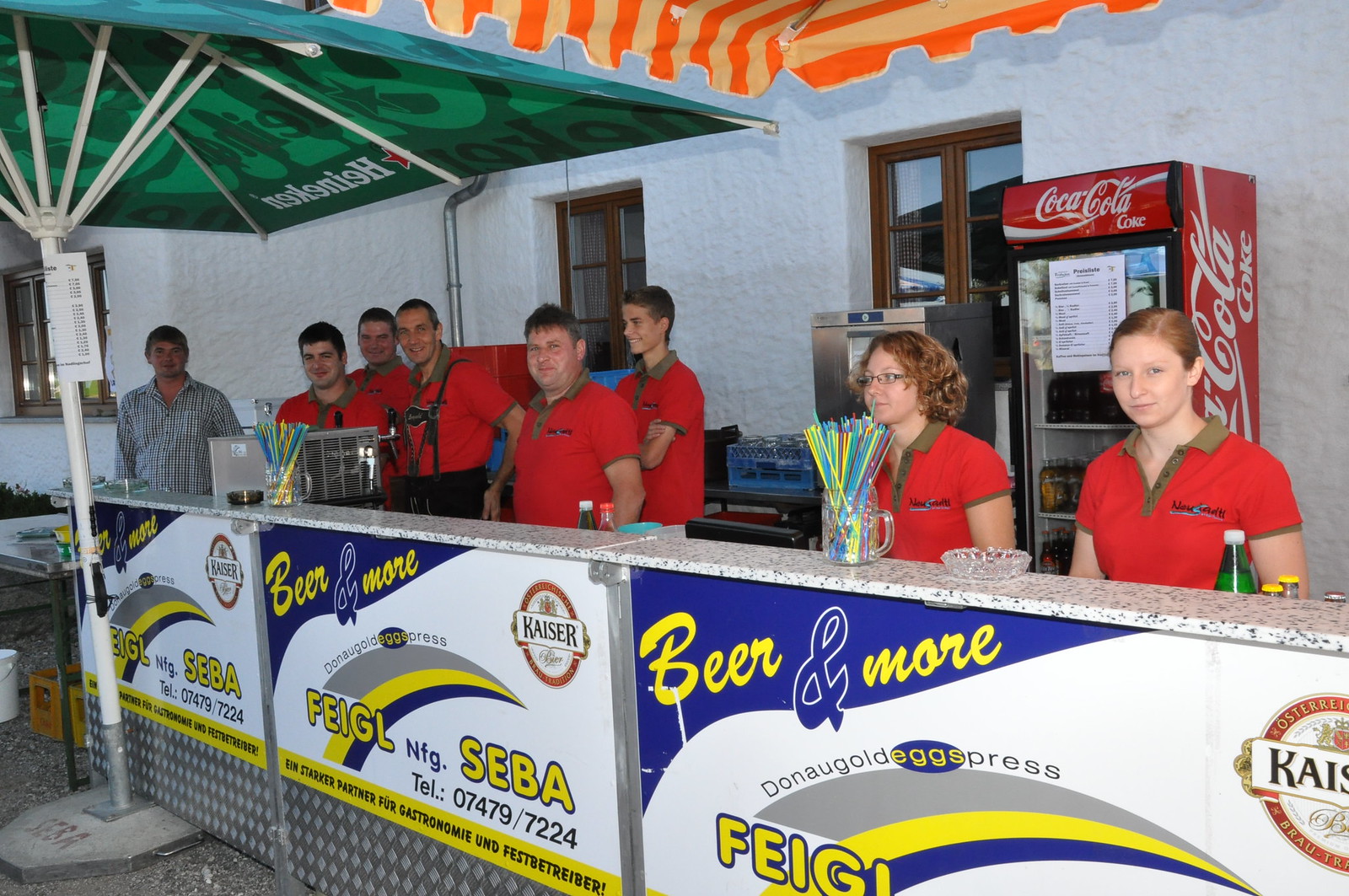This photograph captures a vibrant outdoor makeshift bar constructed from metal fencing material, prominently featuring a large Heineken umbrella that provides shade. The scene is bustling with a group of eight employees lined up behind the bar, seven of whom are dressed in red polo shirts with beige collars, while one person at the far left sports a checkered button-down shirt. Each shirt has a logo on the right-hand side, though the text is not fully legible. The bar itself is adorned with an eye-catching blue banner that reads "Beer and More" in yellow letters, along with additional signage in a foreign language. The banner further displays a telephone number: 07479/7224. Behind the bar staff, a Coca-Cola refrigerator stocked with drinks stands against a white painted wall of a building. On the bar counter, there is a glass mug filled with multicolored straws and a glass ashtray. The environment around the bar showcases a bit of greenery on the left-hand side, reinforcing its outdoor setting. All the employees are facing the camera, posing cheerfully for the photograph.